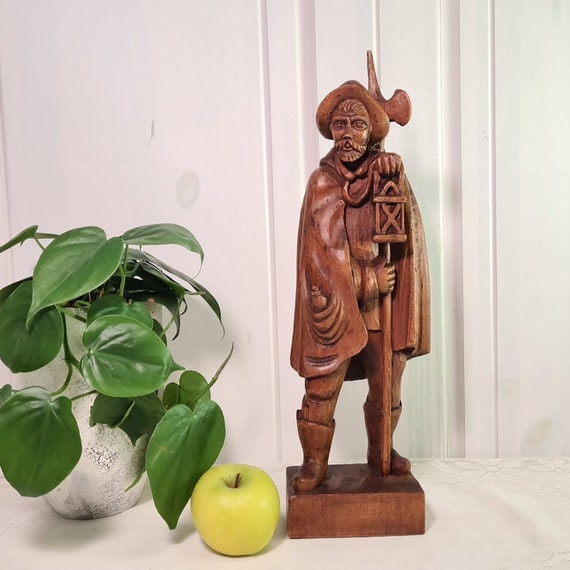This indoor photograph centers on a detailed wooden statue depicting an old-fashioned explorer or swashbuckler-like figure. The statue, about 8-12 inches tall, stands on a small wooden platform and features intricate details such as a large cloak, thick boots, a floppy hat, and a lantern in one hand. The figure also appears to be holding a long, pointed staff or stake, suggesting he might be equipped for a journey or navigation. Behind him, an axe or similar equipment is visible. To the lower left of the statue is a real green apple, resembling a Granny Smith but without any stickers. Further to the left, there's a white stone cylindrical vase containing a potted plant with thick, waxy, spade-shaped green leaves, indicating a healthy, ornamental indoor variety. The backdrop comprises a white, possibly wooden, wall with a table pressed against it, adorned with what appears to be a lace tablecloth, enhancing the domestic setting of the image.